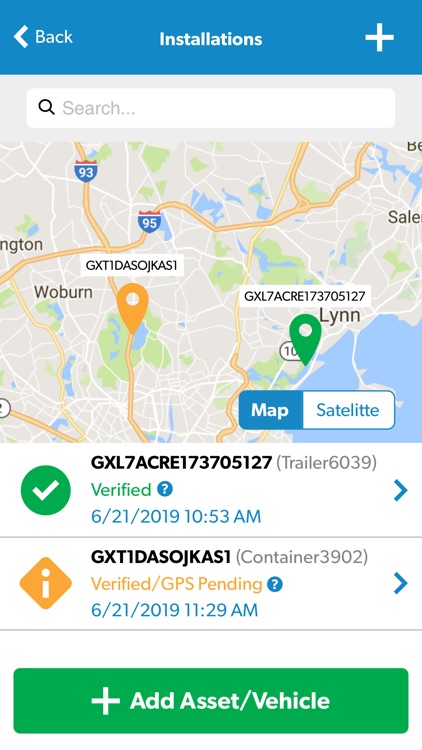The image illustrates a mobile app interface displayed on a mobile device. At the top of the screen, there is a blue navigation bar. On the left side of this bar, a white back arrow is accompanied by the word "Back" also in white. Centered in the bar, the word "Installations" appears in white text. On the right side, a white plus symbol is visible.

Beneath the navigation bar is a map interface. At the top of the map, there's a white search box with a black search button. Within the map, there are two white boxes featuring alphanumeric codes. Additionally, the map includes a yellow location marker and a green location marker. The green marker is labeled as "Verified," while the yellow marker indicates "Verified GPS Pending."

Below the map, there are two tabs that provide more information about the locations associated with the green and yellow markers. Users can click on these tabs to expand the details. At the bottom of the screen, a prominent green button with white text and a white plus icon reads "Add Asset or Vehicle."